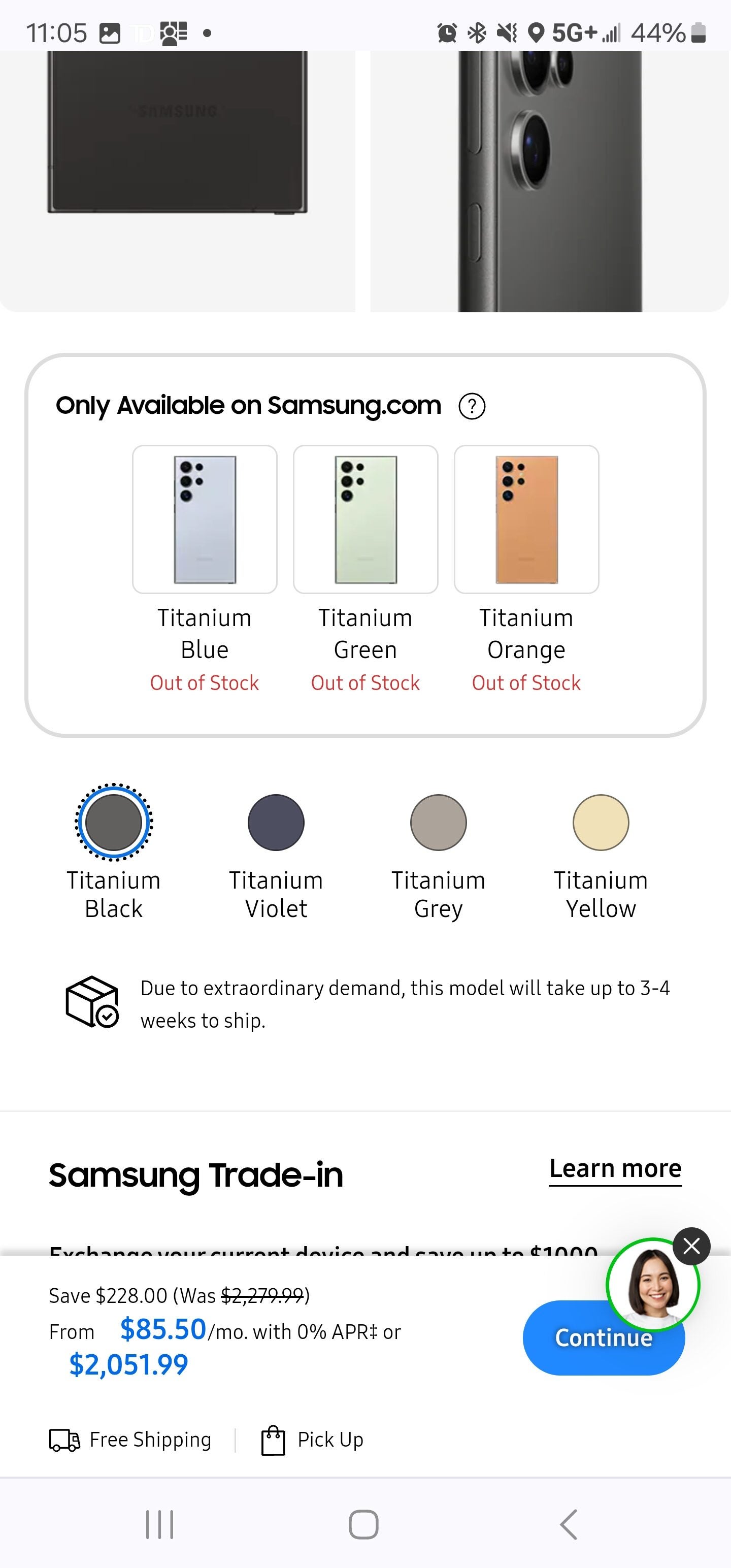This detailed caption is cleaned up for clarity and elaboration:

---

The image is a screenshot taken from a smartphone displaying the Samsung website against a white background. At the top of the screen, the time is shown as 11:05, although the AM or PM indicator is not visible. In the upper right-hand corner, the battery icon indicates it is charged at 44%. Below the header, a partial image of a smartphone is visible on the upper right side.

Underneath this section, there is a rectangular area with rounded edges outlined by a gray line on a white background, showcasing the headline, "Only Available on Samsung.com." This area contains illustrations of the back of three smartphones in different colors, each labeled with their respective color names and availability statuses.

- The first smartphone, labeled "Titanium Blue," is marked as out of stock.
- The second smartphone, labeled "Titanium Green," is also marked as out of stock.
- The third smartphone, labeled "Titanium Orange," appears more gold than orange and is similarly marked as out of stock.

At the very bottom of the screen, the text "Samsung Trade-In" is displayed with "Learn More" next to it, underlined, suggesting a hyperlink. Further down, there is a small circular image showing the head of a woman with shoulder-length brown hair. To the left of this image, the total price of the phone is displayed as $2,051.99. To the right, a prominent blue button labeled "Continue" is visible.